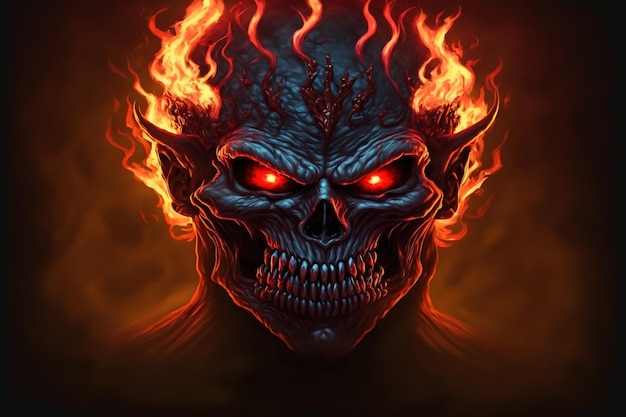This detailed painting portrays a menacing monster or demon figure, centered within a burnt orange-brown background accentuated with black highlights. The creature's head is prominently displayed, featuring a metallic blue skull with a texture reminiscent of a lizard's skin. Most striking are its three rows of shiny, dark metal teeth grimacing menacingly and glowing red eyes that seem to pierce through the viewer. Its skull-like face includes sharply defined, elf-like pointed ears and lacks a nose, showing only the skeletal holes typical of a skull. A fiery mane of orange, red, yellow, and gold flames erupts from the top of its head, creating an ominous aura or halo effect, which illuminates the dark, shadowy surroundings. Dark red, splotchy V-shaped and squiggly designs appear on its forehead, some seeming almost like streaks of dried blood. Additionally, you can glimpse part of its neck, which retains a bit of flesh. The corners of the image dissolve into pitch black, emphasizing the chaotic, fiery aura of the creature. The overall effect is a chilling, dark, and malevolent presence that dominates the image.